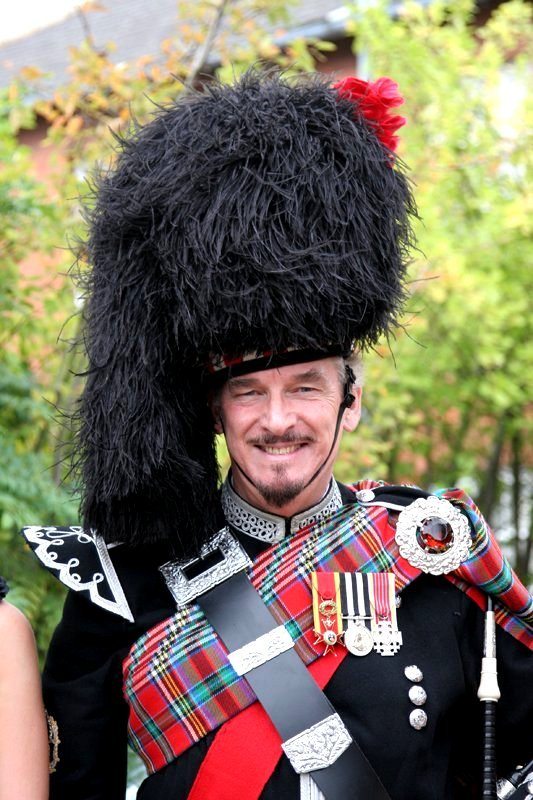In this outdoor daytime photograph, a gentleman is dressed in formal Scottish military attire, reminiscent of a Scottish guard or soldier. He wears a striking tall black hat, made of feathers, that droops to his left side and is adorned with a red ribbon. His black jacket is complemented by a vibrant plaid tartan sash draped across his shoulder, displaying a pattern of red, green, and blue that symbolizes Scottish heritage. His chest is decorated with three military medals and various other pins and buttons. Notably, his left shoulder features a large, ornate silver shoulder pad embellished with a stunning gem. The gentleman is smiling, showcasing his pride in the traditional and distinguished ensemble.